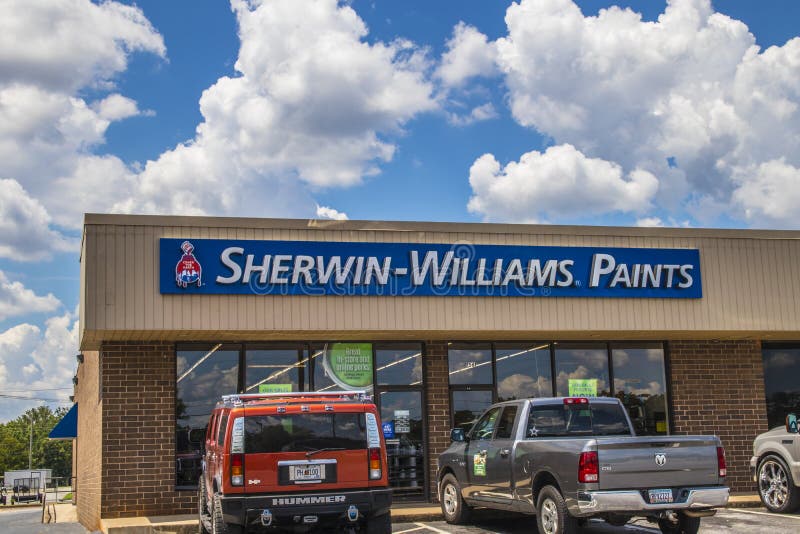A picturesque scene features a tall building with "Sherwin-Williams Paints" emblazoned on it in blue, standing majestically under a sky transitioning from white clouds to a serene blue. The building showcases wooden paneling and brickwork, with large windows that offer a glimpse into the store’s interior. Prominently displayed on one of the central windows is a circular sticker. To the left side of the image, a massive, red Hummer with a metal license plate stands out, showcasing its bulkiness. Nearby, a gray Ram truck with a sleek silver bumper is parked, its wheels partially visible against the backdrop of cement and brick. The scene is speckled with various other objects, contributing to the rich, urban texture of the environment.